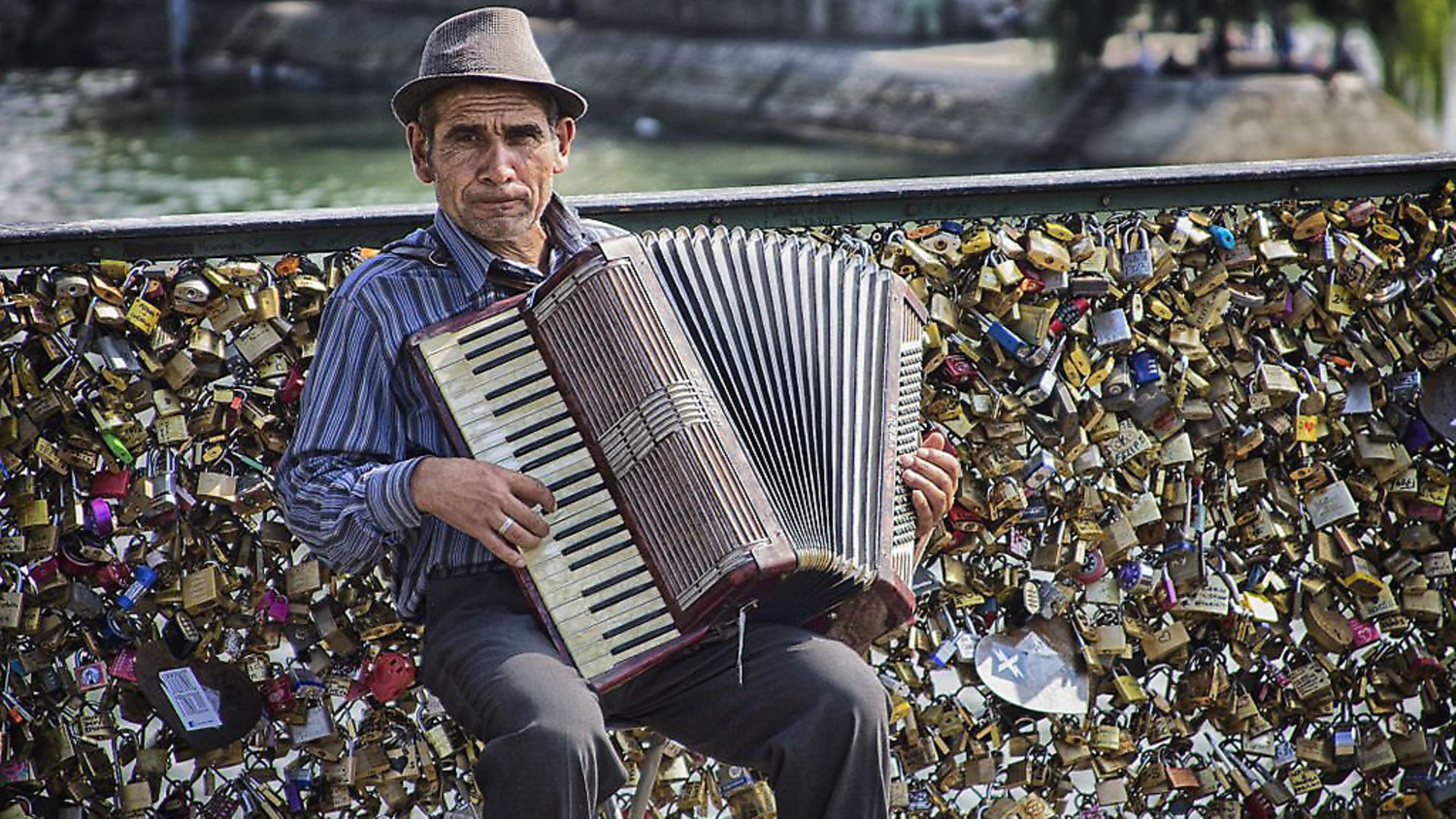In this captivating photo, a man, likely in his 50s, is seated on a small folding chair in front of a bridge heavily adorned with padlocks, symbolizing love. Wearing a gray fedora, a striped blue and white button-down shirt, and grey slacks, he is focused as he plays a large accordion, with his left hand on the chords and his right hand on the keyboard. His lips are pursed in concentration as he looks off to his right. Behind him, the bridge's wire railing is completely obscured by thousands of padlocks hung on the metal rungs, creating a dense, colorful wall of locks. The setting, possibly Venice, allows for a glimpse of water and a portion of a cement area in the upper right corner of the background, further enhancing the romantic and picturesque atmosphere of the scene.